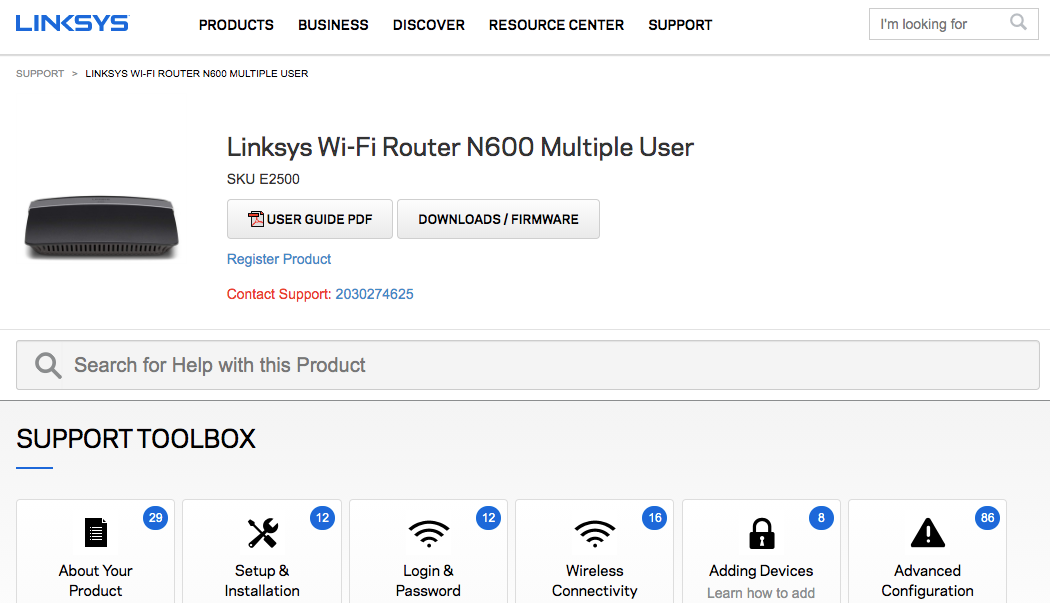At the top left corner, in bold blue capital letters, the text reads "Linksys." To the right, in smaller black letters, are the navigation options: "Product," "Business," "Discover," "Resource Center," and "Support." Near the right side, adjacent to a magnifying glass icon, there's a text box labeled "I'm looking for...". A gray horizontal line separates this section from the rest of the page.

Below this line, the page is labeled "Support" followed by a series of nested labels: "Linksys," "Wi-Fi Router," "N600 Multiple User." The main header reaffirms the product description with the text "Linksys Wi-Fi Router N600 Multiple User SKU: E2500." 

To the left, there is a small, indistinct picture of the product, colored in black with no discernible features due to its size. 

Beneath the image, there are two gray buttons labeled "User Guide PDF" and "Downloads/Firmware." Under these buttons, in blue text, there is a link that says "Register Product," followed by a red text link that says "Contact Support." Additionally, to the right, there is a blue hyperlink labeled "2030274625."